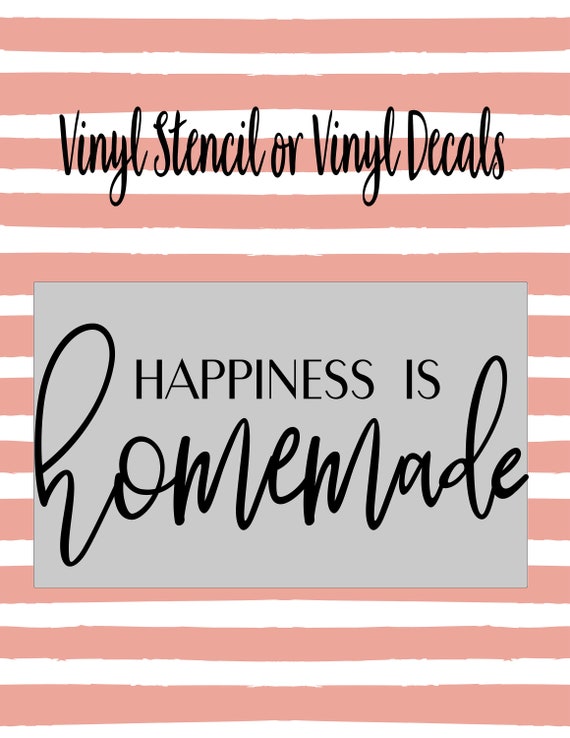The image likely intended for social media or an advertisement showcases a creative design featuring vibrant horizontal salmon (or peach)-colored and white stripes as the background. At the top, in a distinctive handwritten cursive black font, the text reads "Vinyl Stencil or Vinyl Decals." Centrally placed over this striped background is a light gray rectangle. Inside this rectangle, the message "HAPPINESS IS" is written in clear, all-capital black letters, while directly below it, the word "HOMEMADE" appears in the same handwritten cursive style as the top text. This visually appealing layout, combining different font styles and a contrasting background, makes it a compelling and eye-catching design likely used for a business promoting vinyl stencils or decals.